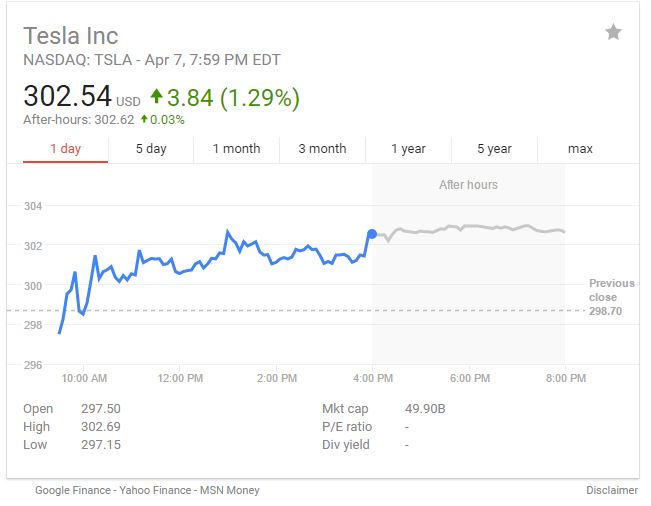The image displays a detailed stock quote for Tesla as of April 7th at 7:59 p.m. Eastern Standard Time. At market close, the stock was valued at $302.54, having risen by $3.84, or 1.29% for the day. In after-hours trading, the stock value slightly increased to $302.62, showing an additional gain of 0.03%, equivalent to $0.08.

The one-day chart highlights Tesla’s stock performance, illustrating its initial value somewhat close to $298. Throughout the trading day, the stock experienced fluctuations, eventually stabilizing and steadily inclining to the closing value of $302.54 at 4 p.m. The after-hours activity remained relatively flat with a marginal rise of $0.08.

For additional reference:
- The previous close was $298.70.
- The opening value was $297.50.
- The highest value of the day was $302.69, while the lowest was $297.15.

The stock quote also displays a market capitalization of nearly $50 billion, but does not provide a P/E ratio or dividend yield. Various options for viewing the stock's performance over different periods—such as 5-day, 1-month, 3-month, 1-year, 5-year, and maximum—are also available.